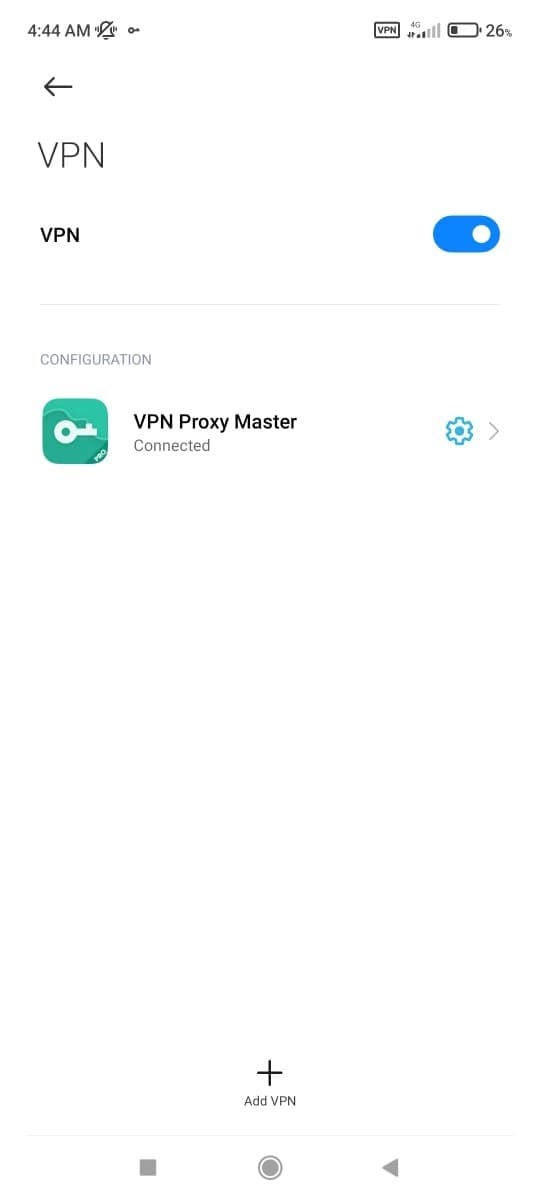Screenshot details from a cell phone display:

- **Time Display**: The screen shows the time as **4:44 AM**.
- **Status Indicators**: To the right of the time, there are indicators for **VPN**, **4G**, and **Battery Life** at **26%**.
- **Navigation Arrow**: Below the status indicators, there is a **left-pointing arrow**.
- **VPN Text & Toggle**:
  - The word **VPN** is presented in all capital letters.
  - Below this, a smaller, bold version of **VPN** is displayed.
  - Adjacent to this text, there is a toggle switch that is currently turned **ON**.
- **Configuration Section**:
  - A very thin white line separates the above elements from the next section.
  - The word **CONFIGURATION**, written in gray and all capital letters, follows.
  - Below this is an app icon featuring a key and split-screen design in two shades of green.
  - The app is labeled **VPN Proxy Master Connected**.
  - Next to this label, there is a **blue gear icon** and a **light gray arrow** pointing to the right.
- **Bottom Section**:
  - At the bottom of the screen, there is a **plus sign** with the label **Add VPN**.
  - Following this, there are three solid shapes in sequence: a **circle**, a **square**, and a **triangle**.

This detailed screenshot offers a wealth of information on the phone's VPN setup and status, encapsulating various UI elements related to configuration and connectivity options.